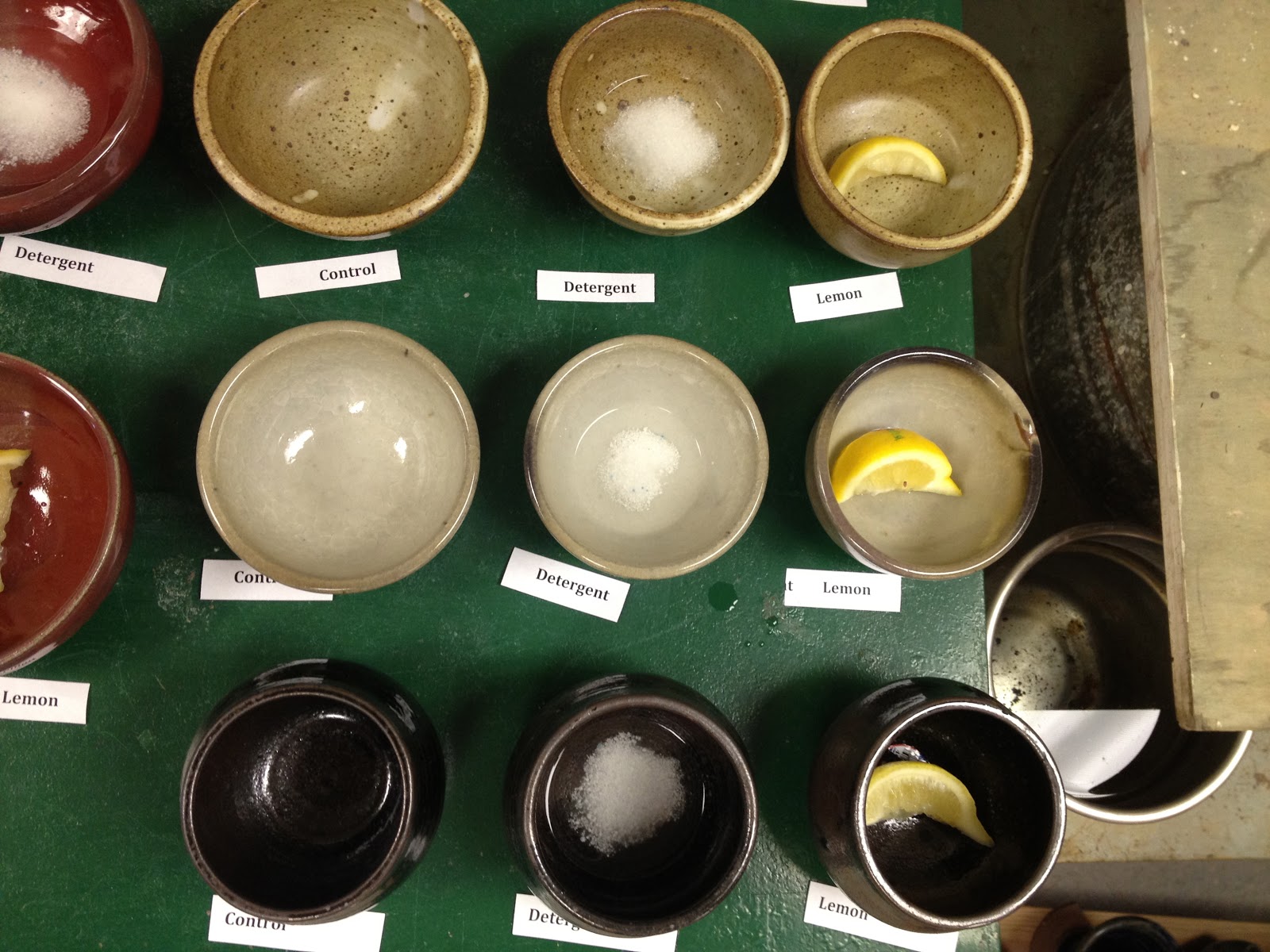The image depicts a green table set up for what appears to be an experiment. Arranged on the surface are several ceramic bowls of varying colors and textures, including lighter shades of gray, reddish hues, and solid dark browns. The bowls are cup-sized and lack handles. They are systematically labeled with paper name tags indicating their contents or purpose. 

From left to right, at the top row, there's a bowl labeled "detergent" containing a flaky, white substance, followed by a "control" bowl which is empty, another "detergent" bowl, and then a "lemon" bowl containing cut pieces of lemon. This setup repeats in a lower row, with "lemon," "control," "detergent," and another "lemon" bowl. Additional smaller brown bowls are placed at the bottom, mirroring the setup with labels for "control," "detergent," and "lemon."

Accompanying the bowls are metal buckets with water positioned to the right of the arrangement, tying into the experimental context. The overall scene suggests a methodical testing of different substances—detergent, lemon, and a control—potentially to explore their interactions or effects.